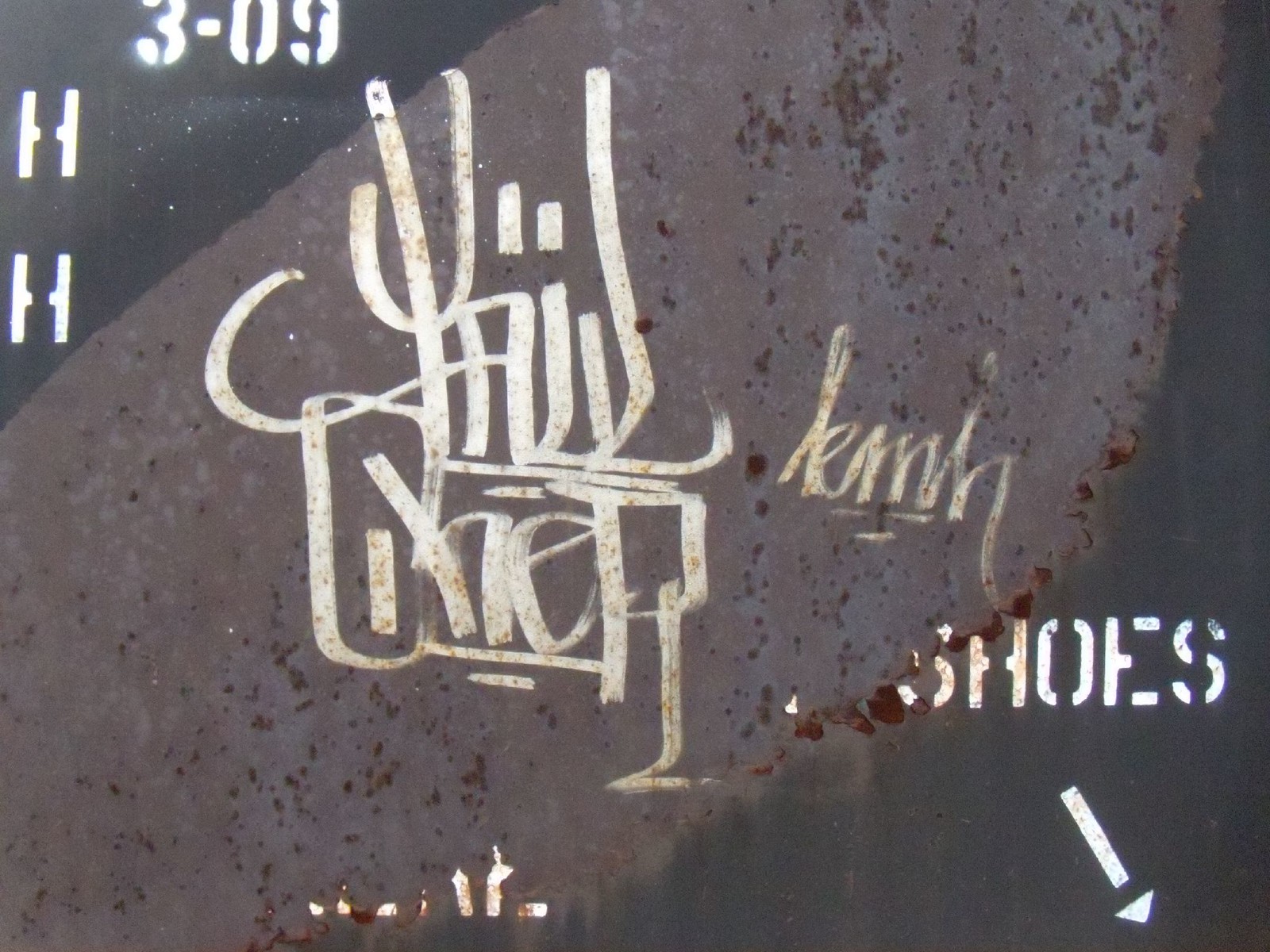This photo captures a graffiti-tagged, weathered metal structure outdoors. The structure, possibly a sign or container, prominently features a large, rusted patch in the center, obscuring its original content. At the bottom right corner, white text ending in "shoes" is accompanied by an arrow pointing down and to the right, suggesting a direction related to shoes. In the top left corner, the numbers "3-09" are clearly visible above two ambiguously interpreted H's, characterized by broken lines through their centers. Over this rusted and faded area, a graffiti tag, potentially signed by an artist named L-E-M-M or similar, dominates the scene in stark white lettering. Beside this main tag lie additional smaller markings, such as "K-M-H," further adding to the layered visual story written in decay and urban artistry.